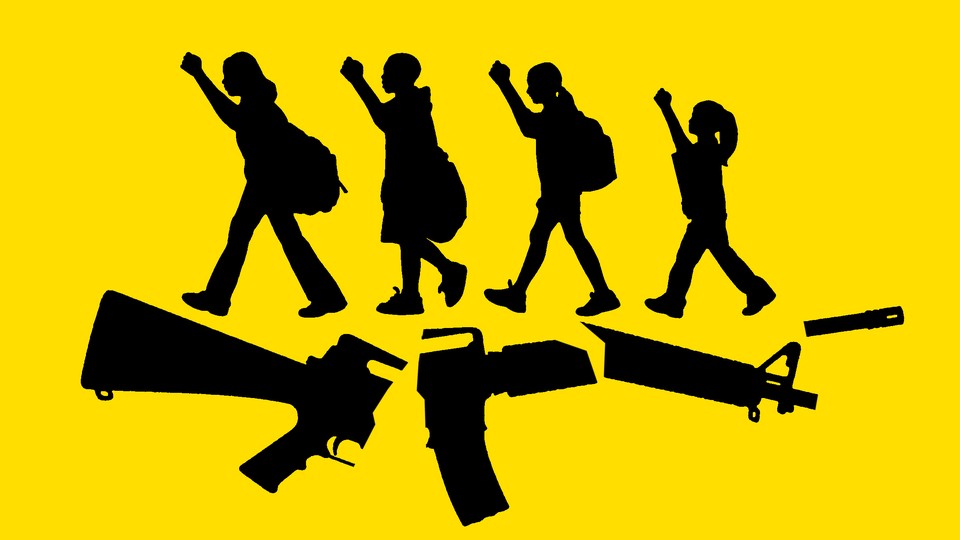The image features a bright yellow background with distinct black silhouettes. At the top of the image, four children are walking from right to left, each with a raised fist. The children appear to be in silhouette, with one girl at the back with a ponytail, followed by another girl with a ponytail and a backpack, then a boy with a backpack, and finally a child whose gender is not clear, also carrying a backpack. The sizes of the children decrease from right to left, indicating a perspective or a movement sequence. Below the children, in the middle and towards the bottom of the image, is a broken assault rifle, likely an AK-47, divided into four pieces. The simplicity and contrast of black against the bright yellow draw attention to the themes of protest and anti-violence, symbolized by children marching above the dismantled weapon.